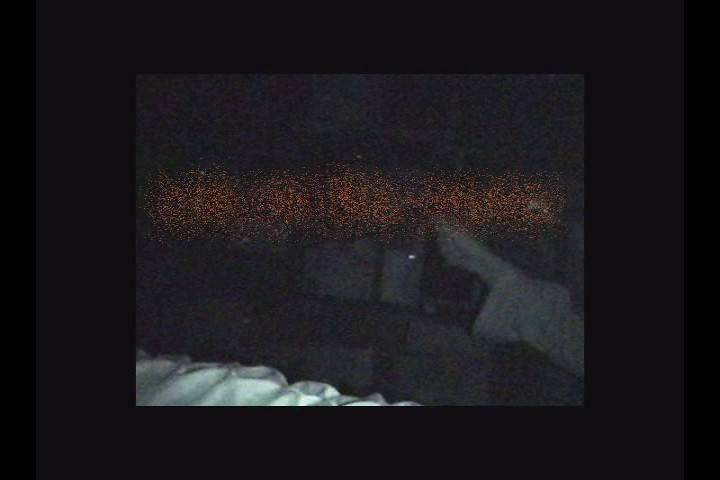A predominantly black image serves as the background, with a solid black rectangle occupying the entire frame. Nested within this is a smaller, dark and blurry rectangle that depicts an indistinct image. Though unclear, a notable feature within this rectangle is a foggy, horizontal orange smear line situated slightly above the center, stretching from the left edge to the right. In the bottom left corner of the smaller rectangle, a white, soft-looking object is visible, possibly a sheet or blanket. On the right side, an ambiguous form resembling a hand or foot extends across the image, making contact with the orange smear line.